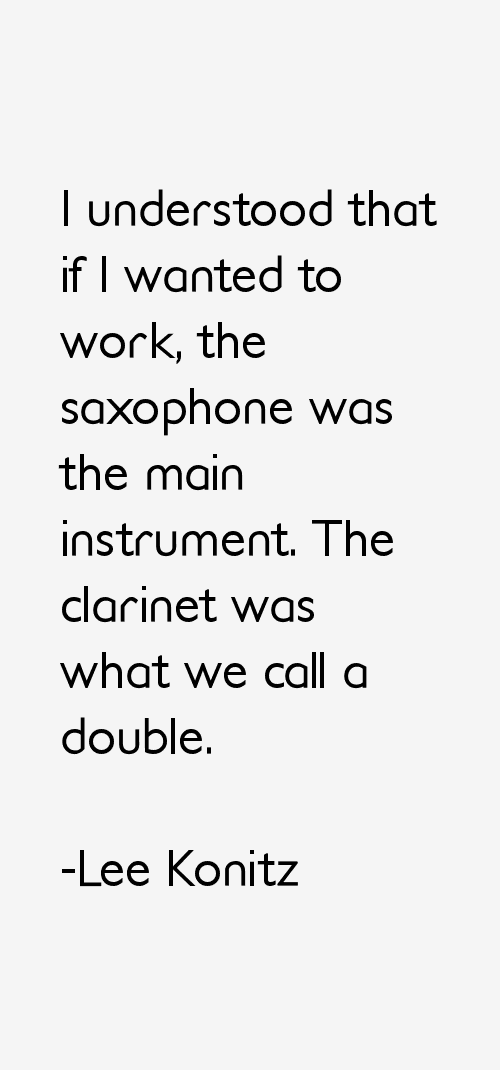The image is a vertically oriented rectangle with a light gray background, featuring a centered quote in standard black text that reads: "I understood that if I wanted to work, the saxophone was the main instrument. The clarinet was what we call a double." Below the quote, there is a dash followed by the name "Lee Konitz." The text is evenly spaced, with larger margins at the top and bottom compared to the sides, giving it a balanced and clean appearance.